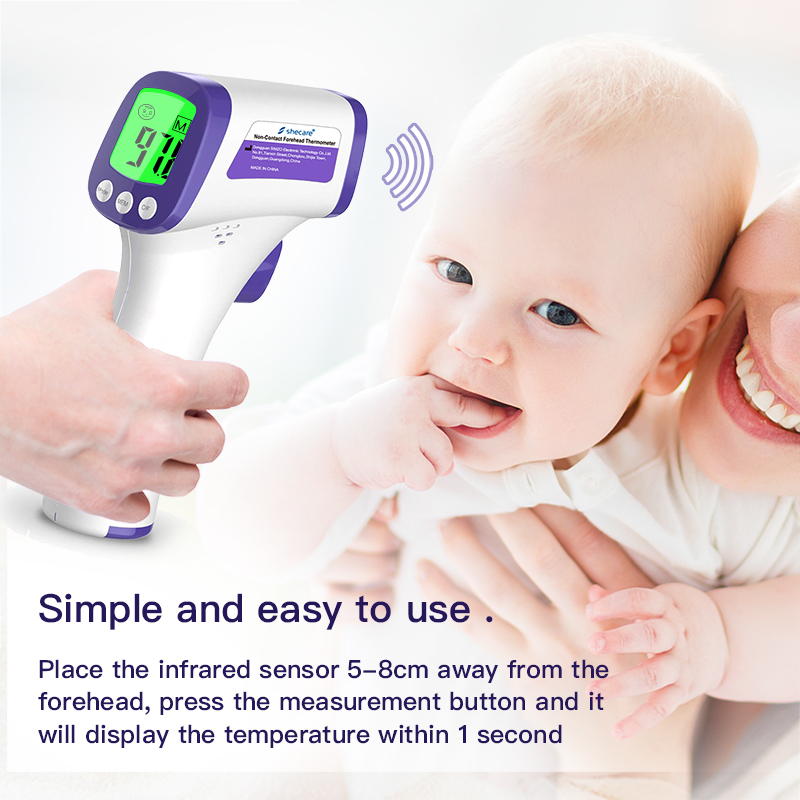The photograph captures the joyful moment of a smiling baby with bright blue eyes and fine reddish-blonde hair, happily sucking on its fingers. Dressed in a white onesie, the baby is cradled by its mother, whose partial face is visible, highlighting her perfect white smile. The baby's chubby hand adds to the endearing scene. From the left side of the photo, a right hand extends into the frame, holding a white and blue infrared thermometer aimed at the baby's forehead. The thermometer's display reads 97.8, indicating its function. Adjacent to the thermometer, an illustrated sound wave directs towards the baby's head, emphasizing the action being performed. At the bottom of the image, blue text provides clear instructions: "Simple and easy to use. Place the infrared sensor 5 to 8 centimeters away from the forehead, press the measurement button, and it will display the temperature within one second." The overall composition suggests it is likely an advertisement for the infrared thermometer.